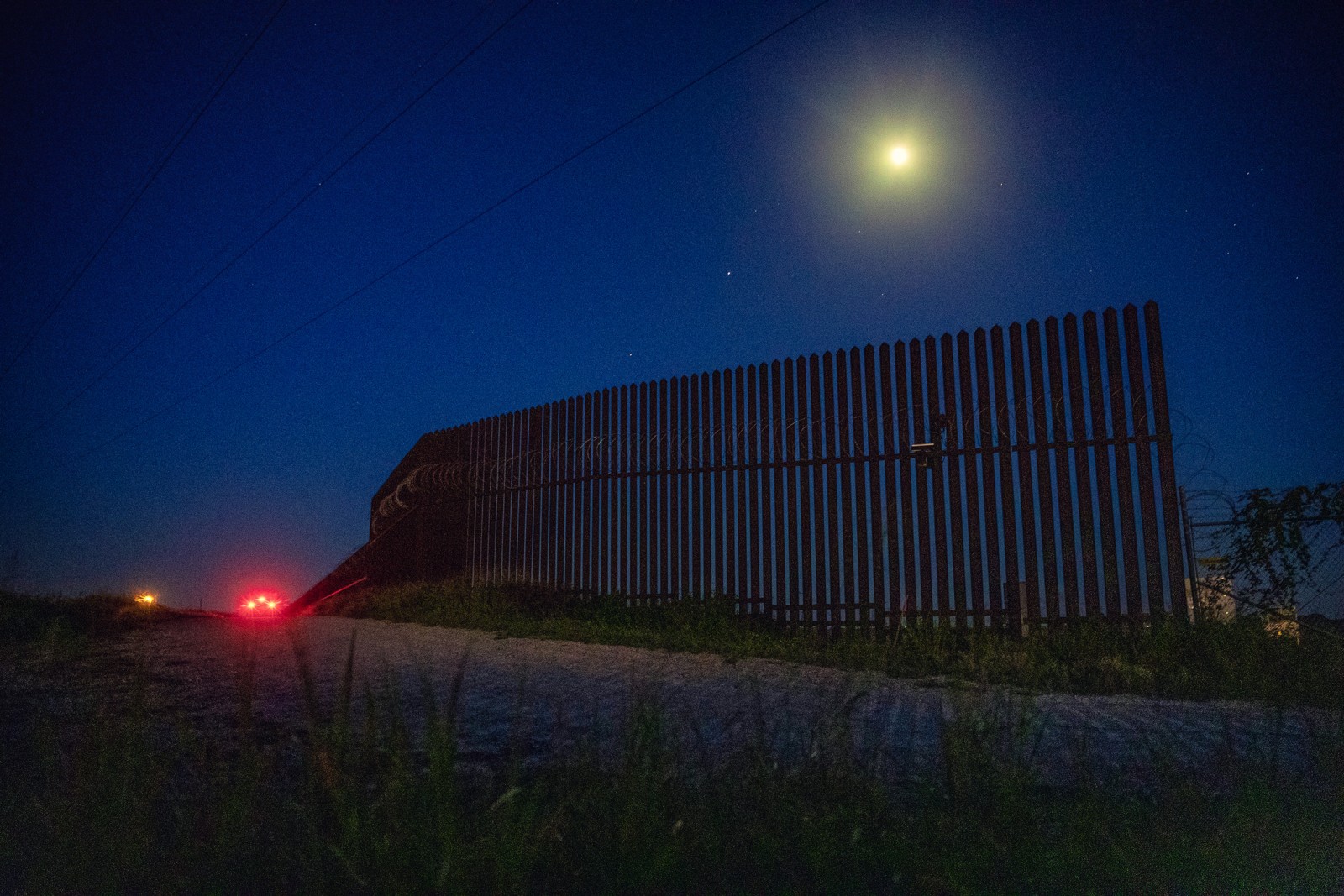The image depicts a tall, imposing fence resembling a border wall, standing prominently under a deep, midnight blue sky. The fence is constructed from closely placed vertical posts, connected by horizontal crossbars and topped with barbed wire, adding to its formidable appearance. In front of the fence, there stretches a road flanked by patches of grass and sparse shrubs interwoven with vines. Along the right side of the fence, there's an additional layer of chain link fencing. Two cars are visible on the road; one car’s red taillights suggest it is moving away from the camera, while another car's orange-hued lights face the camera. Above, the bright moon illuminates the night sky, which is also dotted with faint stars. In the distance, a few buildings with illuminated windows stand against the backdrop of the clear sky, and three power lines can be faintly seen in the upper left corner, adding an extra layer of detail to the stark, eerie scenery.